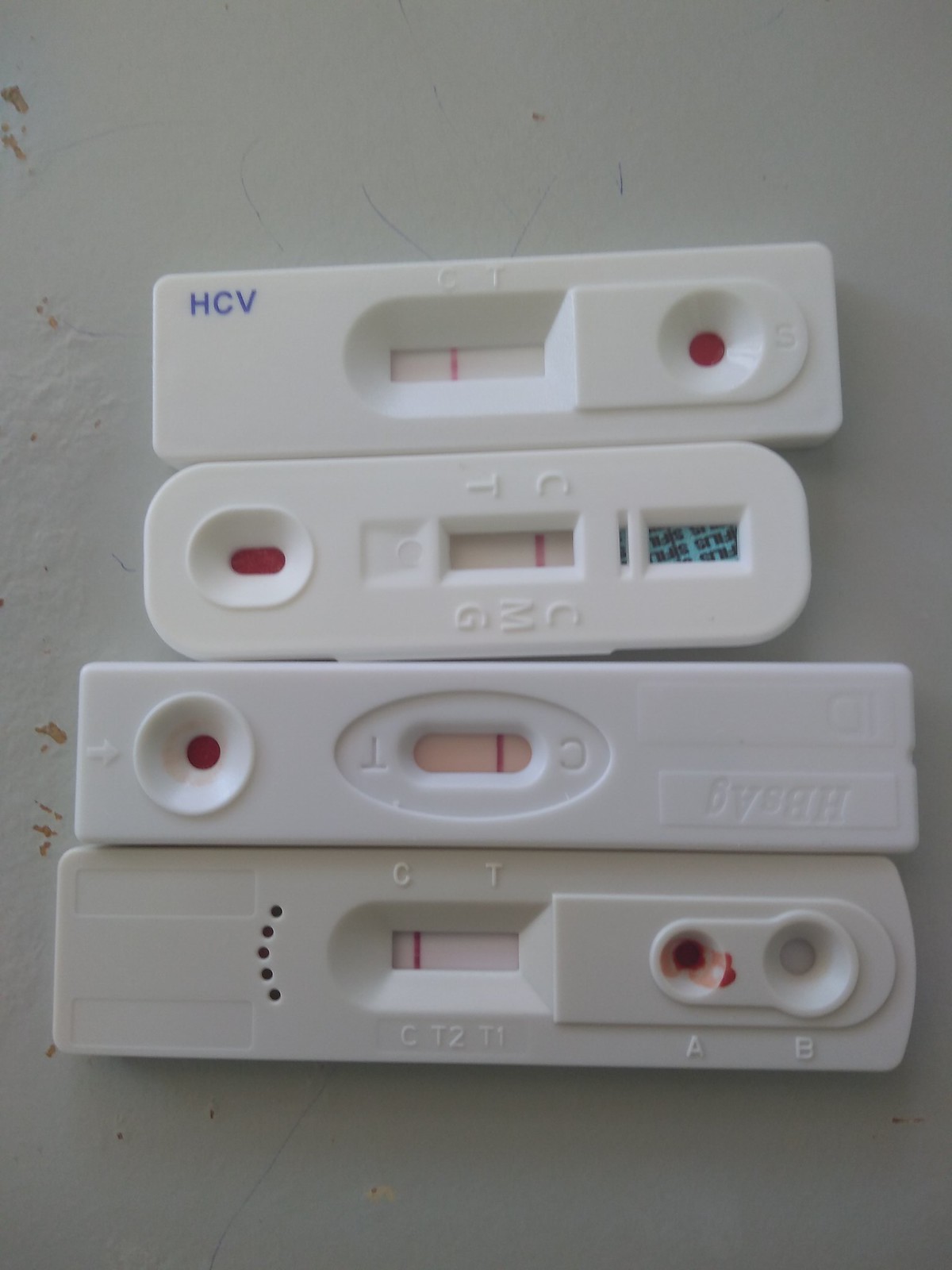The image showcases a series of test kits arranged side-by-side on a stained table, which appears particularly marred on the left-hand side. Each test kit has distinctive characteristics:

1. The first test kit is chunky, displaying a visible line next to the letter "C" but with no marking next to the letter "T." The "A" section of this kit exhibits some staining with a red substance that might be blood, while the "B" section remains clean.
   
2. The second test kit is somewhat less boxy and is whiter in color. It features a solid line near the letter "C" within a circle, although this marking is subtle and requires close inspection. This kit also shows a reddish, blood-like stain within the circled area.

3. The third test kit is noticeably smaller, with a line across the letter "C" and a solid red area inside an oval-shaped section.

4. The final test kit is labeled "HCV," with a faint line running across the "C" next to the "T" and a reddish stain inside the circled section.

The test kits rest on a table that, although not filthy, appears visibly unclean.